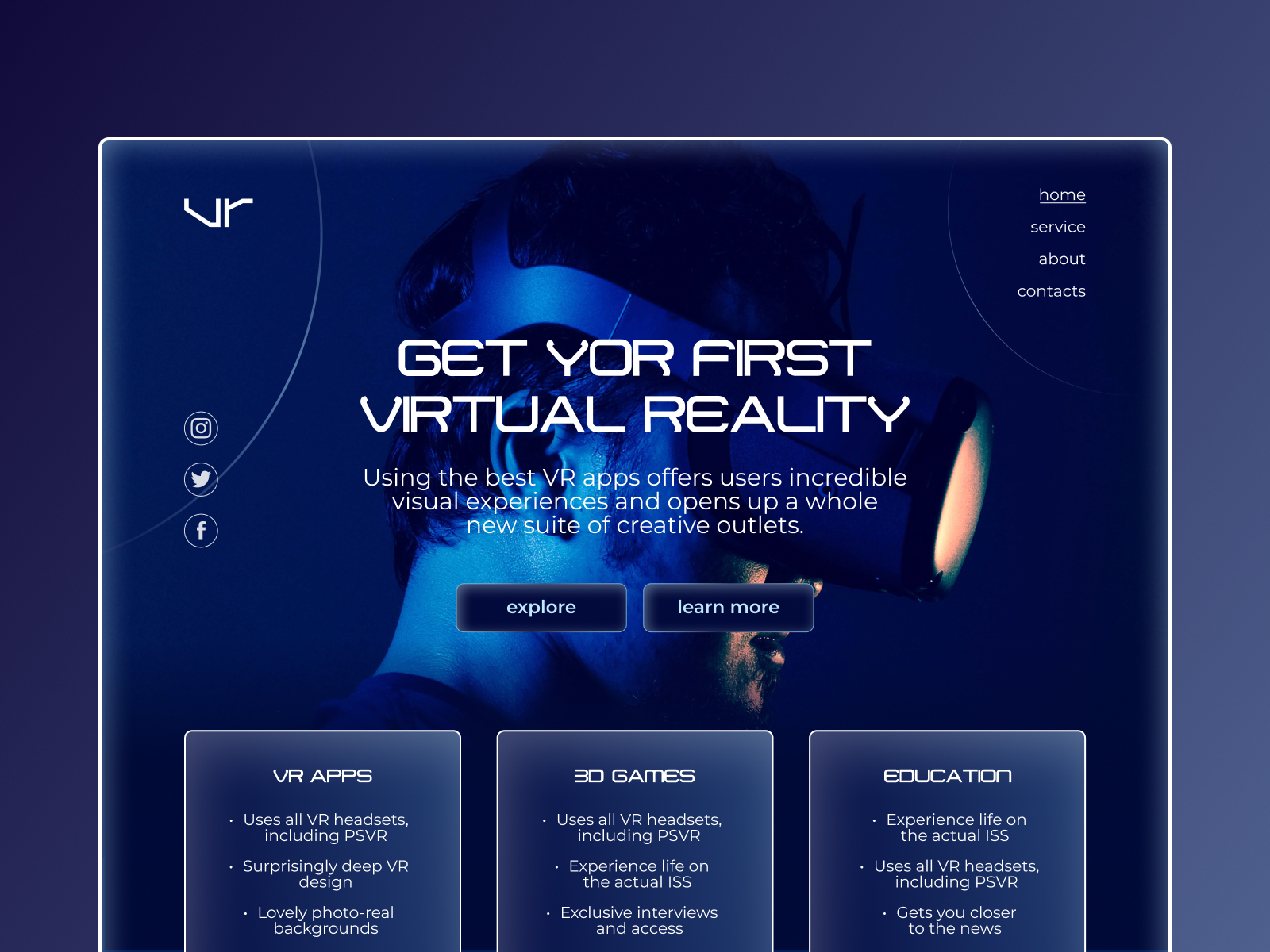The image features a dark blue background with a prominent white outline square in the center. In the top left corner, the initials "VR" are written in white. On the top right, a navigation menu lists options: Home, Service, About, and Contact, all in white text. Center-left, three social media icons for Instagram, Twitter, and Facebook are also depicted in white. 

In the center of the square, a headline reads "Get your first virtual reality," followed by a description stating: "Using the best VR apps offers users incredible visual experiences and opens up a whole new sort of creative outlet." Below this, two dark blue buttons labeled "Explore" and "Learn More" are displayed.

The background image features a person wearing a VR headset, facing the right side. At the bottom of the image, three text boxes provide further information:

1. The first box on the bottom left, titled "VR apps," notes: "Use all VR headsets including PSVR. Surprisingly deep VR design. Lovely photoreal background."
2. The middle box titled "Creative Games" states: "Use all VR headsets including PSVR. Experience life on the actual ISS. Exclusive interviews and access."
3. The bottom right box, titled "Education," mentions: "Experience life on the actual ISS. Use all VR headsets including PSVR. Gets you closer to the news."

Each text and element is cohesively presented in white, maintaining visual harmony against the dark blue background.